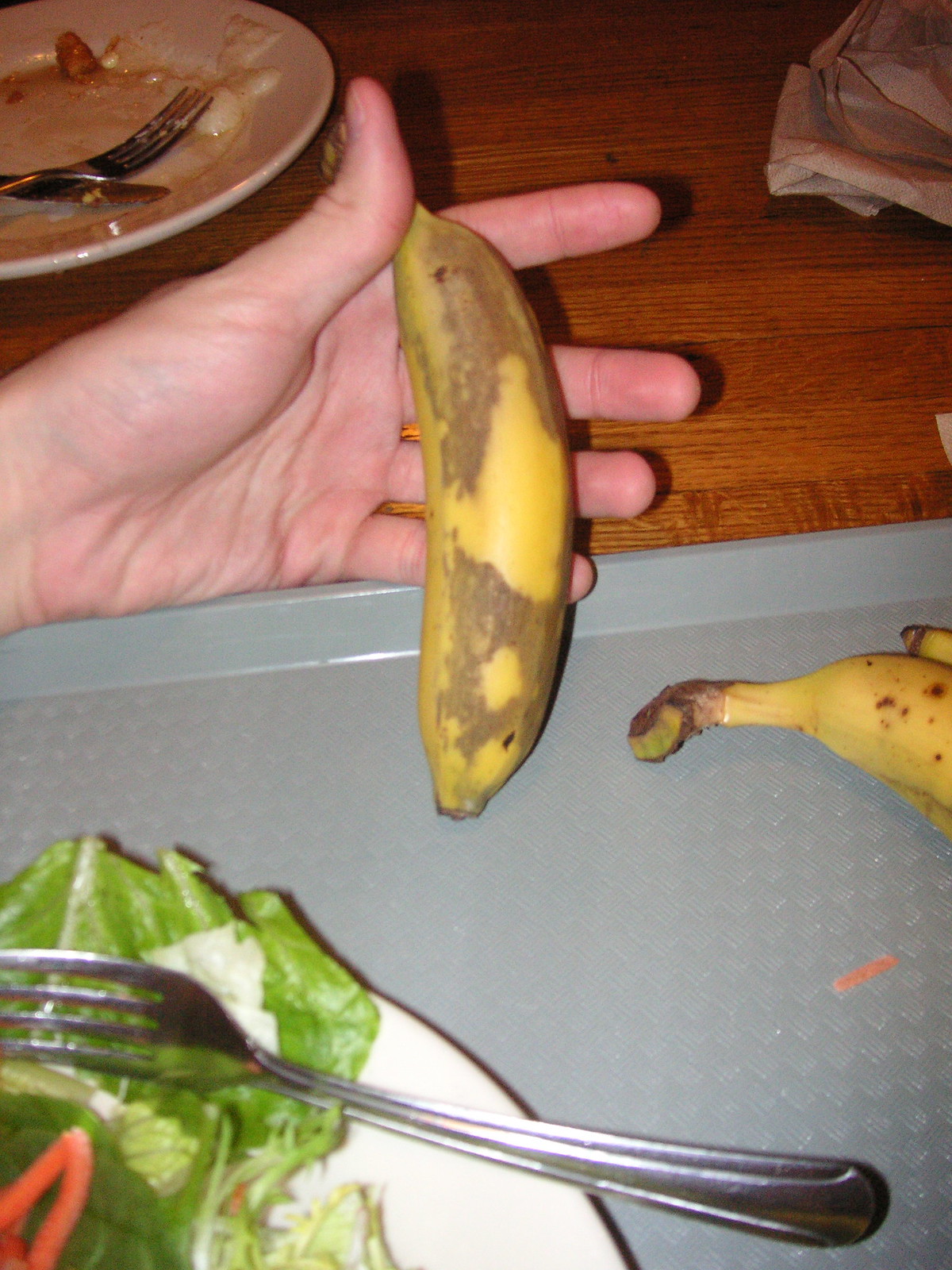In this detailed image, a person is holding a small banana with a slightly brown peel at both the top and bottom, while their palm is facing upward. The banana rests against a gray plastic tray, which partially reveals the tops of two other bananas on its left side. To the right of the tray, there's the edge of a white plate containing a salad composed of lettuce, various green elements, and some kind of tomato. A fork is also visible on this plate. In the background, beyond the person's hand, a wooden surface can be seen with another plate on it. This secondary plate, now empty except for some oily residues and white cream, holds a dirty fork and spoon crossed over each other on its right side. To the left on the wooden surface, brown paper towels or napkins are observable.